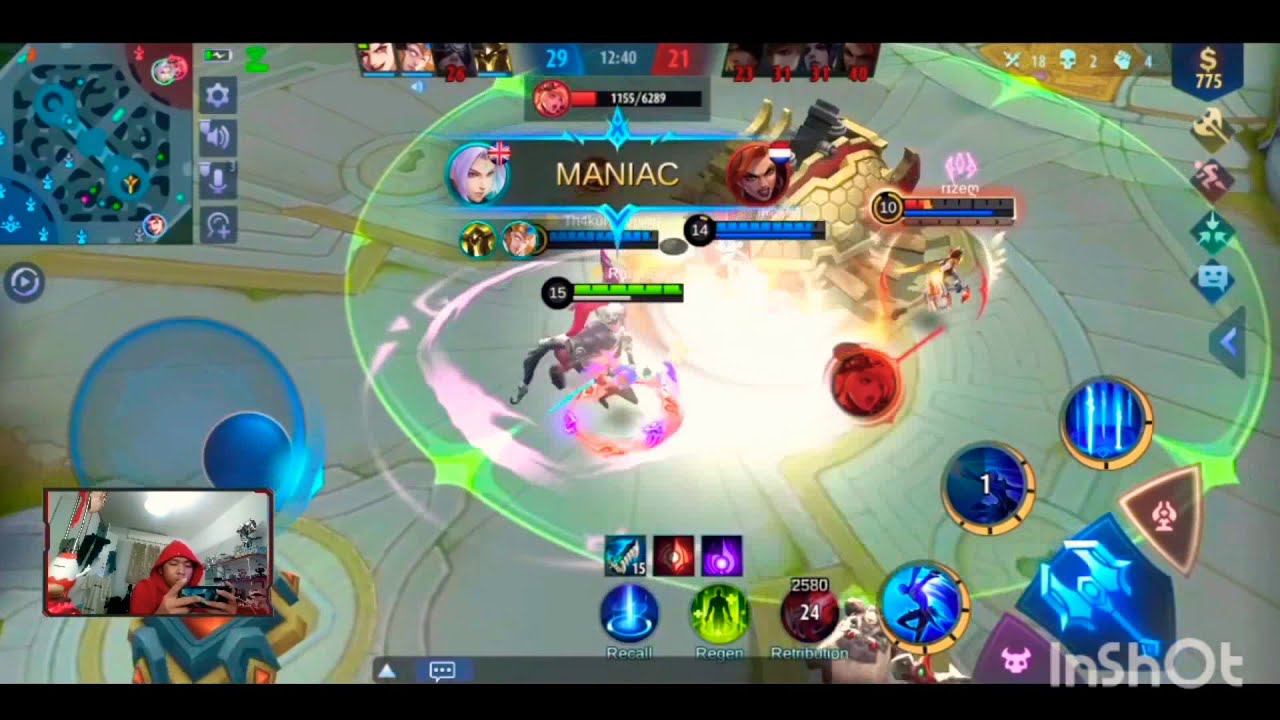The screenshot depicts a vibrant and chaotic video game scene on a monitor. Dominating the screen is a colorful array of shapes—squares, circles, rectangles, triangles—in a myriad of colors including blue, white, orange, green, red, and yellow. At the center of the turmoil is a bright white light encircled by green, with the word "Maniac" prominently displayed above it on a black background. Flanking this word are two characters: a female with purple hair and a British flag to the left, and another with red hair and a French flag to the right. 

Above these characters, the scoreboard reads 29 in blue on the left and 21 in red on the right, with a time of 12:40 displayed between them. The lower right-hand corner contains the text "in shot." In the lower left-hand corner, a smaller rectangle shows the gamer, an Asian individual wearing a red hoodie with the hood up, playing the game on a handheld device. The room behind the gamer is partially visible, adding a personal touch to the intense gaming moment. Icons indicating different attacks and abilities are scattered around, giving the impression of a complex, action-packed game similar to a mobile version of League of Legends. The overall scene is bustling with activity, though the exact gameplay details remain partially obscured due to the bright central light.